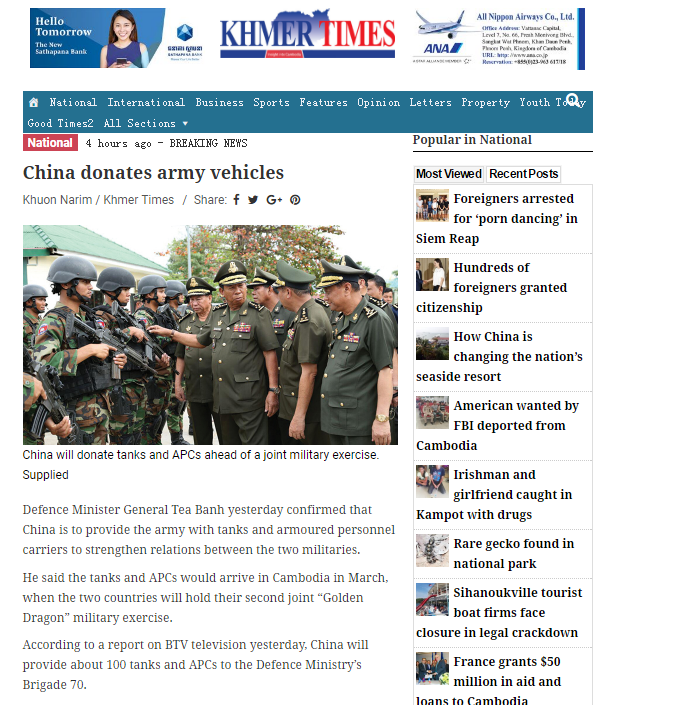This image features an article from the Khmer Times, indicated by the publication's masthead, where "Khmer" is written in blue letters and "Times" in red letters. The layout suggests that it is a military-oriented newspaper. Below the title, there is a blue banner listing various sections including National, International, Business, Sports, Features, Opinion, Letters, Property, Youth Today, Good Times, and All Sections.

At the top-left corner, under a red "National" banner, there is a “Four Hours Ago Breaking News” update. The headline, prominently displayed in black letters on a white background, reads, "China Donates Army Vehicles." The byline credits Khuon Narim from Khmer Times.

The article can be shared on social media platforms such as Facebook, Twitter/X, and Google Plus. 

A photo accompanying the article shows military officers on the right side in dark green dress uniforms with brass buttons and dress hats. On the left, approximately five or six soldiers in camouflage uniforms carry automatic rifles.

Underneath the image, there is a caption stating, "China will donate tanks and APCs ahead of a joint military exercise." The article elaborates that Defense Minister General Tea Banh confirmed China’s donation of tanks and armored personnel carriers (APCs) to fortify bilateral military relations. The tanks and APCs are scheduled to arrive in Cambodia in March for the second "Golden Dragon" joint military exercise. The report, which aired on BTV, mentions that around 100 tanks and APCs will be given to the Defense Ministry's Brigade 70.

To the right of the article, there are links to other news stories:
1. Foreigners Arrested for Porn Dancing in Siem Reap.
2. Hundreds of Foreigners Granted Citizenship.
3. How China is Changing the Nation's Seaside Resort.
4. American Wanted by FBI Deported from Cambodia.
5. Irishman and Girlfriend Caught in Kampot with Drugs.
6. Rare Gecko Found in National Park.
7. Sihanoukville Tourist Boat Firms Face Closure in Legal Crackdown.
8. France Grants $50 Million in Aid and Loans to Cambodia.